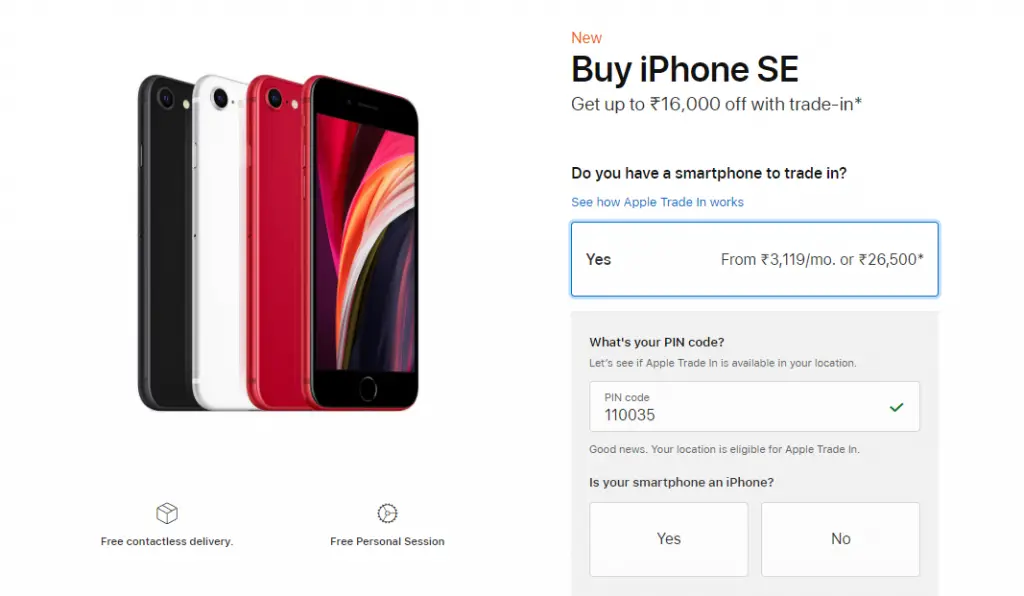The advertisement showcases a clean, white background with a detailed layout of promotional offers for the iPhone SE. On the left, there are images of four cell phones, displaying different colors and views: 

- The first phone is black, shown from the back.
- The second phone is white, also viewed from the back.
- The third phone is red, with the back cover visible.
- The fourth phone is red as well, but it is shown from the front.

Below the cell phone images, there are two promotional snippets:

- "Free contactless delivery," illustrated with an image of a box.
- "Free personal session," accompanied by an image of a camera lens.

The right side of the advertisement features key promotional text on a white background:

- The word "NEW" stands out prominently in red letters, indicating a new listing.
- Below that, in black letters, the offer states: "Buy iPhone SE, get up to $16,000 off with trade-in."

Following this, a question is posed: "Do you have a smartphone to trade in?" with a link below encouraging viewers to "See how Apple trade-in works."

Beneath this, a call-to-action button reads "Yes," with pricing details stating, "from $3,119 a month or $26,500."

Further down, a light gray box prompts for a pin code, saying: "Let's see if Apple trade-in is available in your location." For demonstration, a sample pin code "110035" is used, and the site confirms: "Good news, your location is eligible for Apple trade-in."

Finally, a query asks: "Is your smartphone an iPhone?" with clickable options for "Yes" or "No."

The advertisement is formatted to be engaging and informative, seamlessly guiding the viewer through the promotional details and trade-in eligibility process.